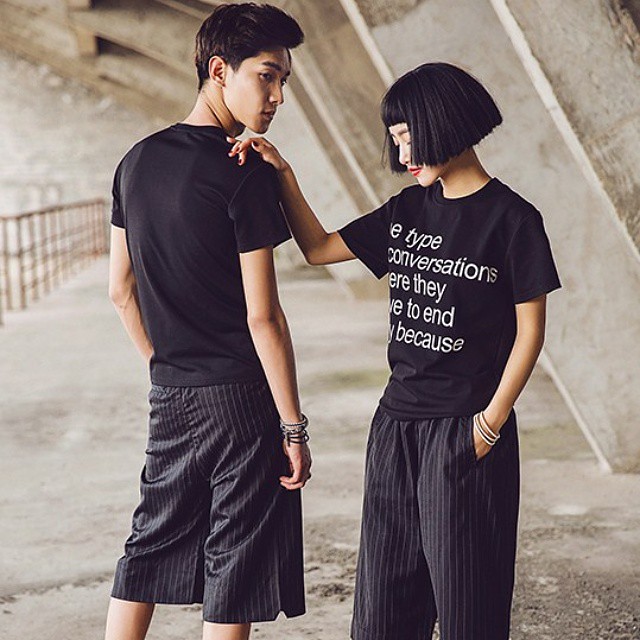The image features two Asian models, a boy and a girl, standing in a concrete alleyway with an arched wall in the background. The boy, positioned on the left, wears a black t-shirt and black shorts with white pinstripes. He stands with his back facing the camera but has turned his head over his right shoulder, revealing the right side of his face, including his eyes and nose. His short black hair is cut just around chin level. The girl, positioned on the right, stands close to the boy, with her right hand resting on his right shoulder. She faces towards us but looks downward, her eyes closed and lips painted with red lipstick. Her left hand is in her pocket. She also sports a short black hairstyle with bangs, and her black t-shirt displays partial text in an aerial-style font, including the words "type conversations they to and because." Both are wearing matching black shorts with white pinstripes and bracelets—his on his right arm and hers on her left.